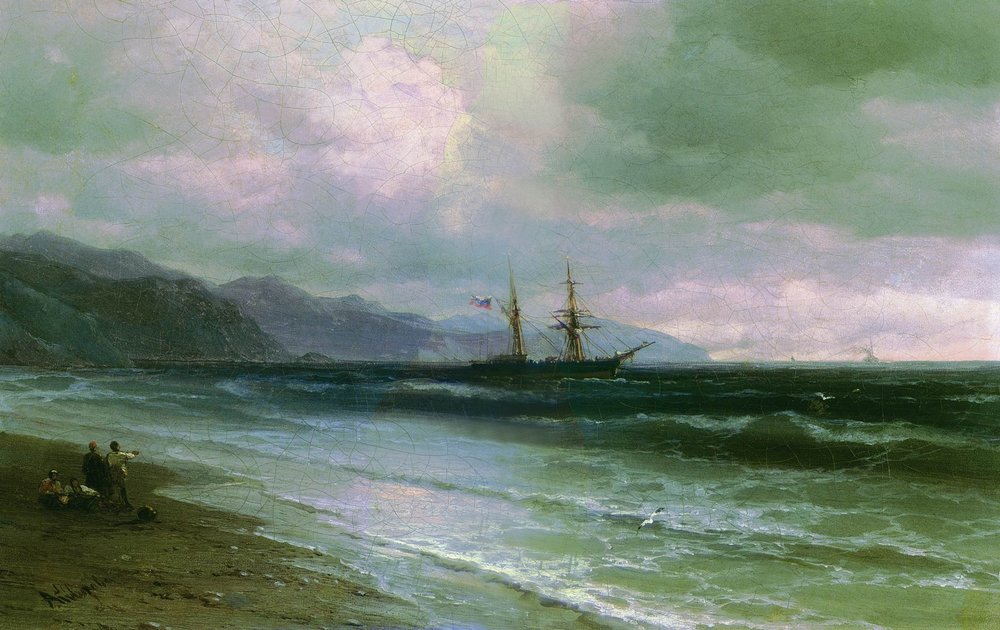This wide, rectangular painting exquisitely depicts an early morning or possibly late afternoon seashore scene. Dominating the composition, a long, dark gray schooner with two large masts rests in the center, near the horizon line. The ship proudly flies a blue, white, and red flag, possibly of French origin. The water, painted in varying shades of greenish gray, grows darker and choppier towards the horizon, where it meets a range of gray mountains that fade into the distance.

In the foreground, the seashore at the bottom left corner is composed of dark, greenish-gray sand interspersed with rocks and patches of green grass. A small group of about four people occupies this area; one person, wearing a white shirt, points towards the ship. Two individuals stand while two others sit, all focused on the vessel. This detailed scene is set against a dramatic sky filled with gray, yellow, pink, and purple clouds, hinting at an overcast day with potential rain. The meticulous detailing and harmonious blend of colors make this painting a captivating maritime piece from the 18th or 19th century.